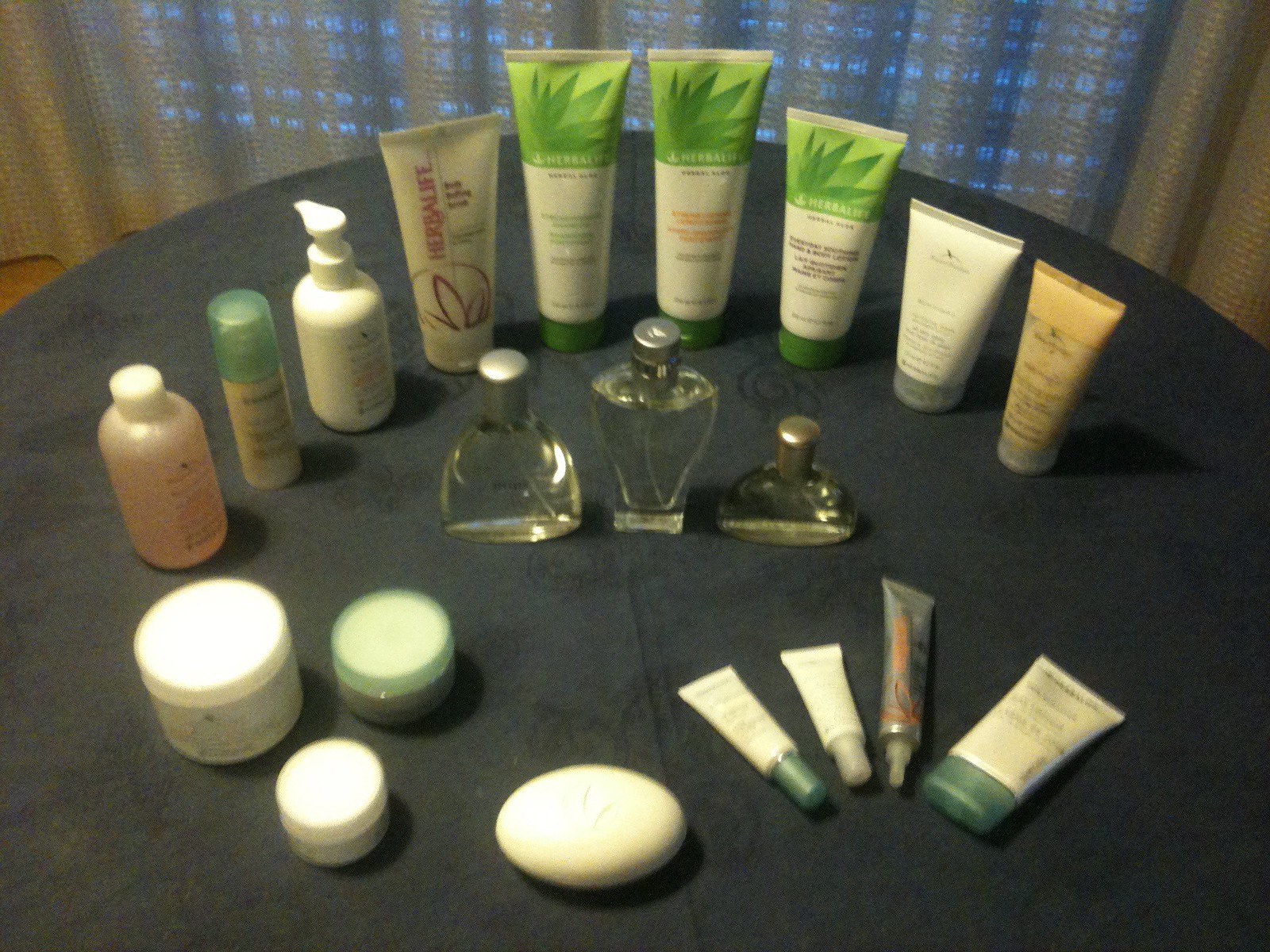On a circular gray table, a diverse array of body and fragrance products is neatly arranged. In the background, an orange curtain partially reveals a wide-hole screen. The ensemble of items includes nine bottles from Herbalife, standing tall in the background. These bottles seem to be a variety of body care products, though their precise purposes are not clearly discernible; one noticeable bottle is outfitted with a pump, likely used for dispensing lotion. Centered on the table are three elegant fragrance bottles. At the forefront, three round canisters with twist-on lids are prominently displayed, accompanied by an unboxed bar of soap. To the right of the soap, four tubes of various products are laid flat on the table, completing the meticulously organized display.